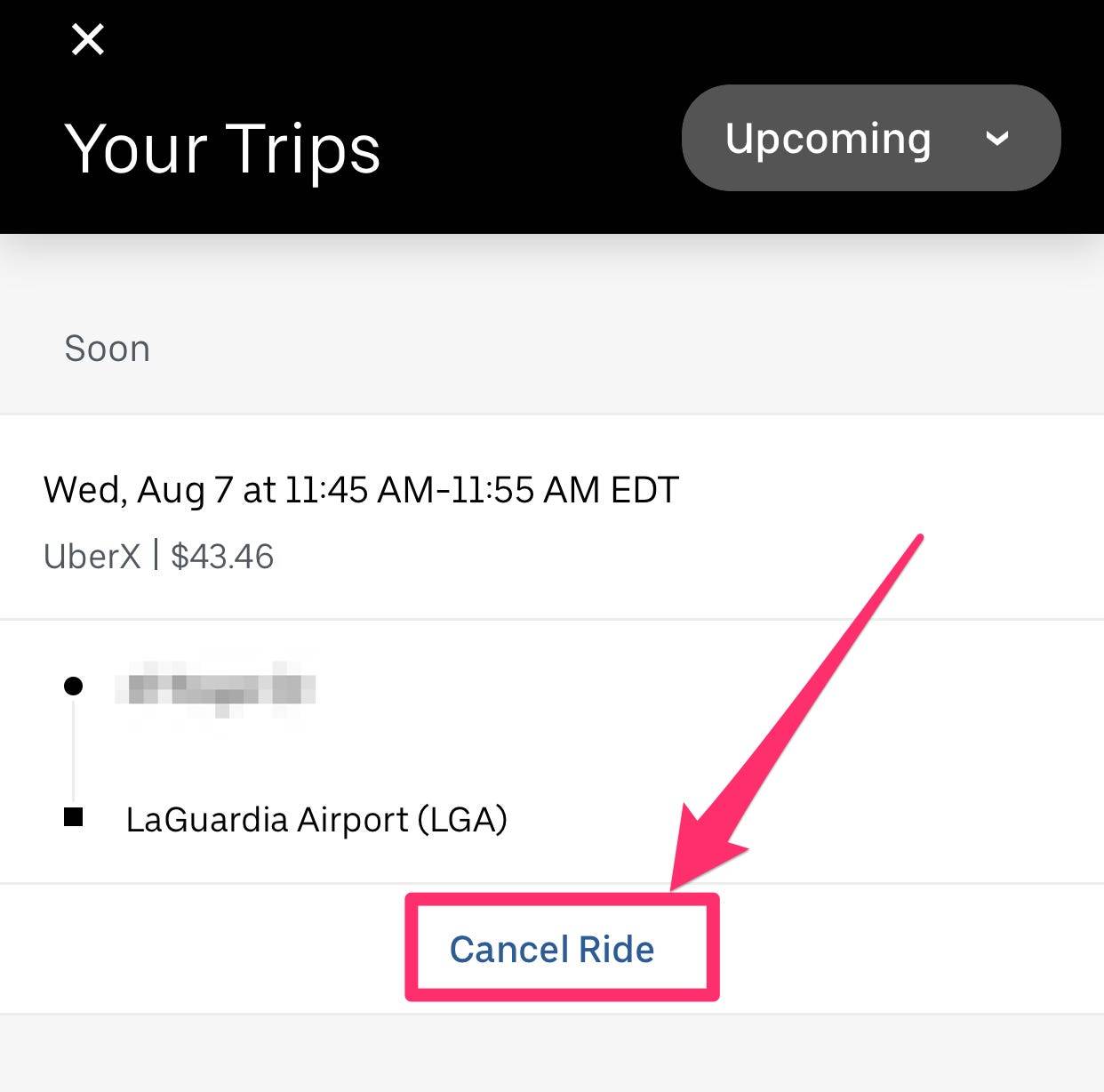The image is a screenshot of a trip management interface. At the top, there is a wide black header featuring a white 'X' icon in the upper-left corner. Directly below the header, large white text reads "Your trips." To the right of this text is a button labeled "Upcoming," accompanied by a pull-down arrow. Underneath this section, a gray banner displays the word "Soon" in gray text. The main content area following this banner has a white background. It provides detailed trip information in black text: "Wednesday, August 7th | 11:45 AM - 11:55 AM EDT." Below this is the fare information in light gray text—"UberX $43.46." A black circle connected by a vertical line to a small black square appears next, followed by a light gray horizontal line. Finally, at the bottom of the interface is a red-outlined button featuring a prominent red arrow and the text "Cancel Ride."